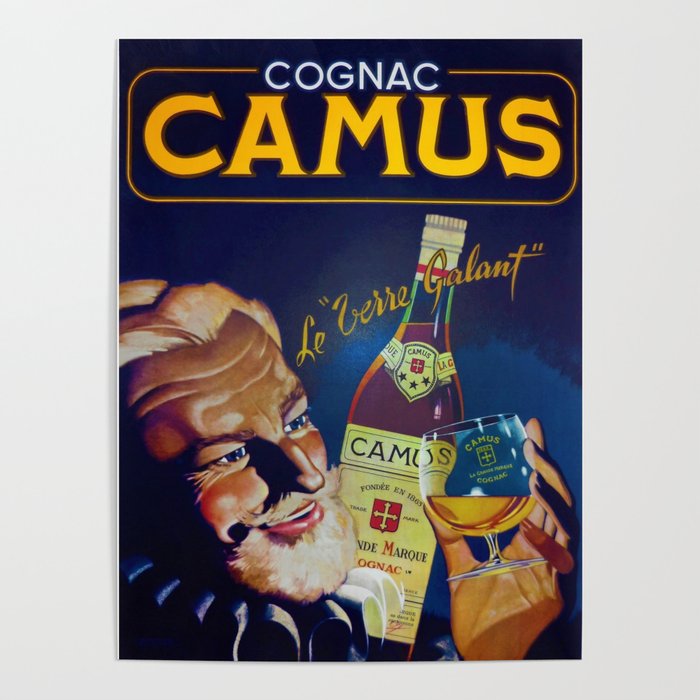This vintage advertisement features a distinguished elderly man with white hair, a white beard, and blue eyes, dressed in a frilly, Elizabethan-style blue and white collar. He is smiling, revealing his teeth. The background is a deep navy blue. The top of the ad displays the word "Cognac" in white text, and "Camus" in larger, bright yellow letters beneath it, both surrounded by an orangey-yellow border with a cutout where "Cognac" sits. The man's left hand is raised, holding a small moon-shaped glass with a yellowish liquid, clearly labeled with "Camus Cognac." Behind him, there is a large bottle of Camus, featuring a white cap and a detailed label with a blue and yellow shield and a red cross. The label includes text that reads "Le Verre Galant" in yellow and a section of it is partially obscured by the man's head. The overall feel of the ad suggests it is from the 1950s or early 1960s, evoking a sense of nostalgia and elegance.